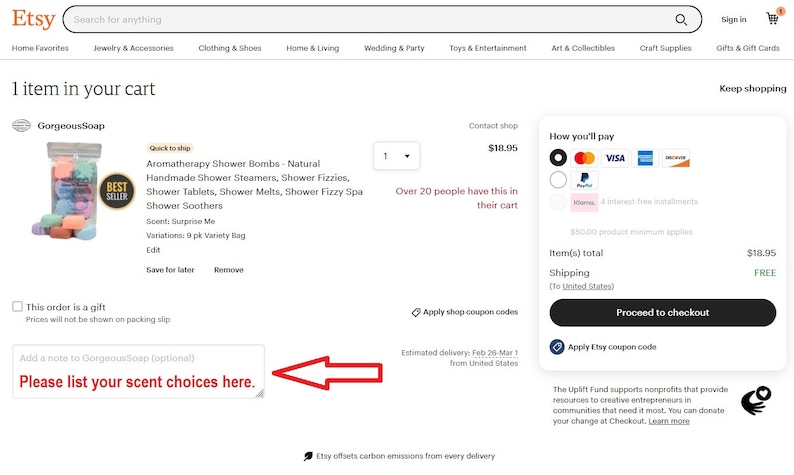This image displays an Etsy store page. In the top left corner, the recognizable orange Etsy icon is prominently positioned next to the search bar labeled "Search for anything" in light gray text. The search bar itself is an elongated black oval with a black border, featuring a magnifying glass icon on the far right. To the right of the search bar are icons for signing in and a shopping cart, which currently has one item in it, marked in orange.

At the top of the page, there's a row of categories including Home Favorites, Jewelry & Accessories, Clothing & Shoes, Home & Living, Wedding & Party, Toys & Entertainment, Art & Collectibles, Craft Supplies, and Gifts & Gift Cards. Directly below these categories, it indicates that there is one item in the cart.

To the left, the product listed is "Gorgeous Soap," which is a bestseller and noted for being quick to ship. The detailed description lists it as an aromatherapy prep item, featuring natural homemade shower steamers, shower fizzies, shower tablets, shower melts, shower fizzy spas, and shower soothers. A note indicates that this order is a gift. Additionally, there is a section for applying shop coupon codes, along with an input section for listing scent choices.

Towards the bottom right, there’s a mention of payment options. The total for the item is $8.95 with free shipping, and a checkout box is located just below this total.